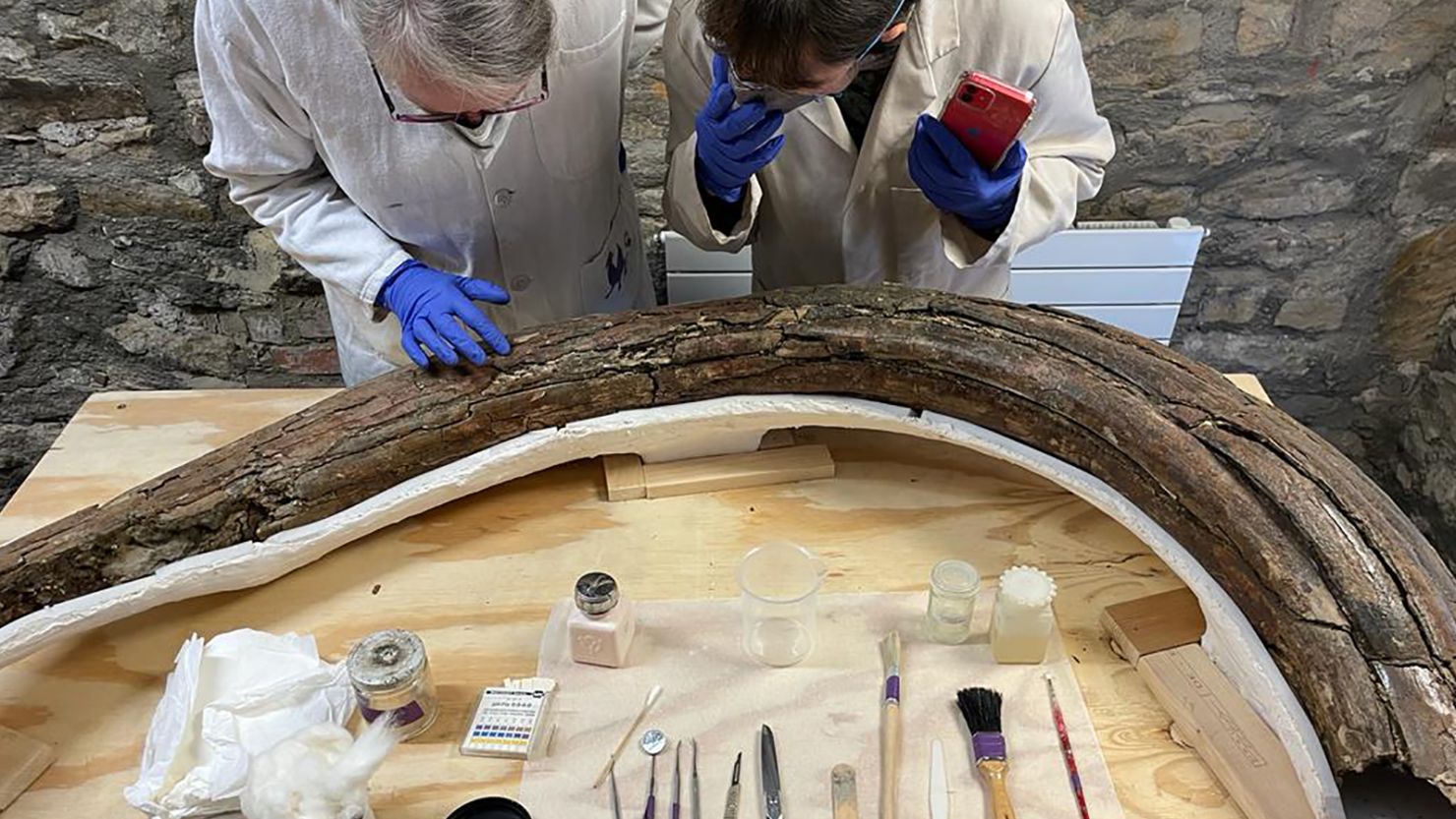In this detailed photograph, two researchers clad in white lab coats and blue gloves are meticulously examining a massive, cracked brown mammoth tusk that is arched in a C formation and placed on a table covered with a neatly organized array of tools and materials. The male researcher, an older gentleman with glasses, focuses intently on the tusk, his hand gently touching its textured surface. The younger, brown-haired female researcher, also wearing glasses, holds a red cell phone in one hand while adjusting a mask on her face with the other. The workspace is meticulously arranged with various instruments, including brushes, jars of liquid, cotton balls, gauze, and small metal objects, all set against a backdrop of a stone wall, creating a precise and engaging scientific investigation scene.